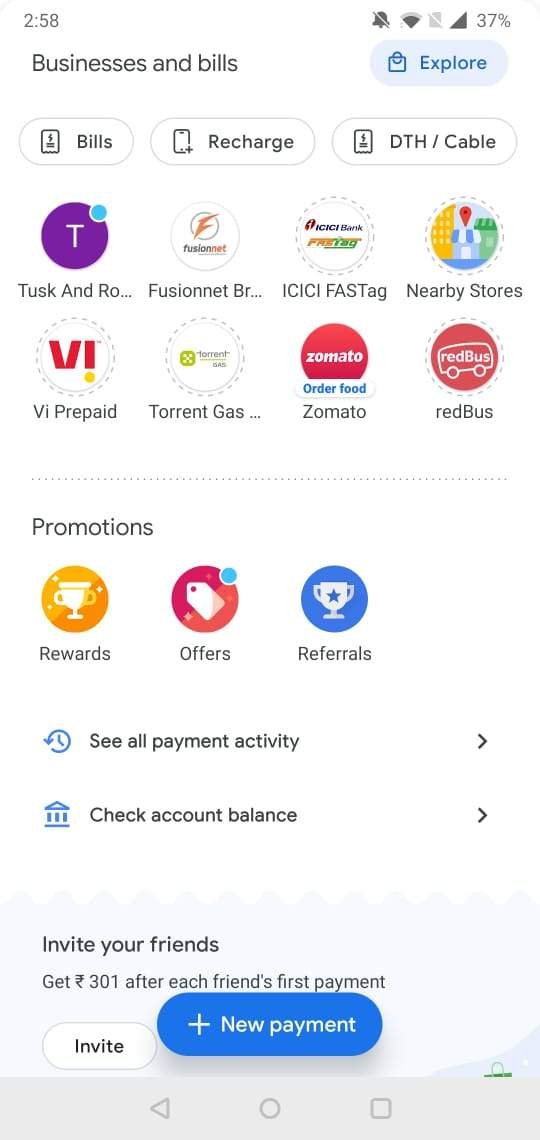The image shows a screenshot of an iPhone display at 2:58 PM, featuring a mobile payment application. The upper right corner displays indicators for reception, ringer status (silent mode), and a battery level at 37%. The main header reads "Businesses and Bills," below which are several functional buttons labeled "Bills," "Recharge," and "DTH/Cable."

Under this section, there are two rows of circular icons representing various businesses and services. The first row includes Tusk, an incomplete name "RO…," FusionNet, ICICI Fast Tag, and an icon for Nearby Stores. The second row features VI Prepaid, Torrent Gas, Zomato, and Redbus.

Further down, there is a section titled "Promotions," with three more circular icons labeled "Rewards," "Offers," and "Referrals." At the bottom of the screen are additional actionable items such as "See All Payment Activity," "Check Account Balance," and "New Payment." This layout suggests that the app functions similarly to Venmo, enabling users to pay for various goods and services directly from their phone.